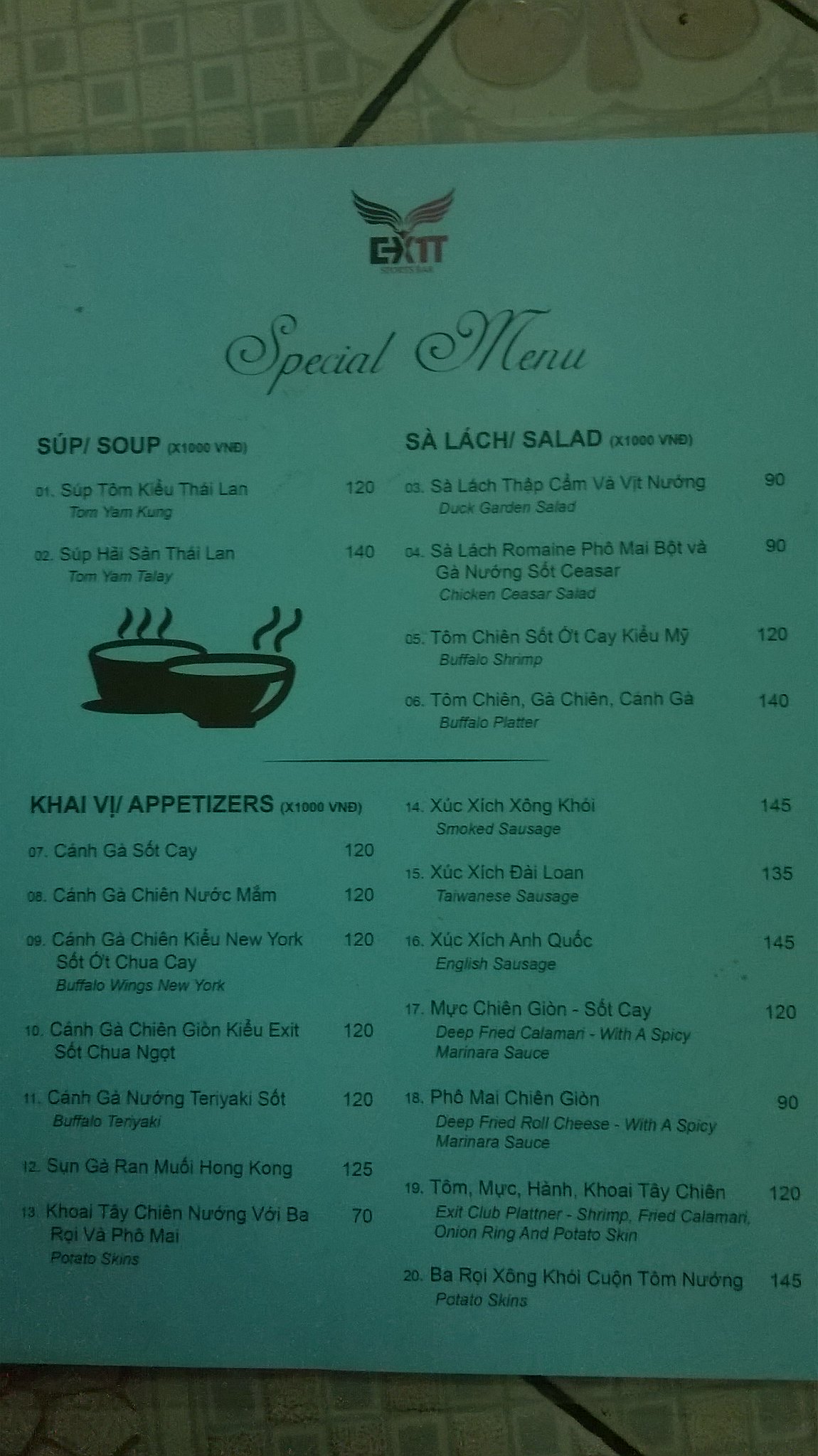The image features a neatly designed menu. At the top center of the menu, the phrase "Special Menu" is elegantly written in cursive. Above this, there's a distinctive logo featuring the word "exit," accompanied by wing-like graphics that are linear, with one side of the wings in black and the other in red.

On the left side of the menu, the word "soup" is written twice, likely indicative of different languages, with two different soup options listed below. These are accompanied by a small black-and-white illustration of a bowl of soup. The menu is densely populated with various items, including appetizers, each listed with a corresponding price not in English, ranging from approximately $1.40 to $1.45.

To the right of the soup section, there is a "Salad" column, offering several different salad options. The entire menu comprises 20 items, each sequentially numbered from 1 to 20. Each dish is followed by a brief description, separated by horizontal lines, providing clarity and structure.

The photograph of the menu has a slightly grayish tint, suggesting a possible filter or lighting condition affecting the color. The layout is well-organized and evenly divided, ensuring a clean and readable appearance.